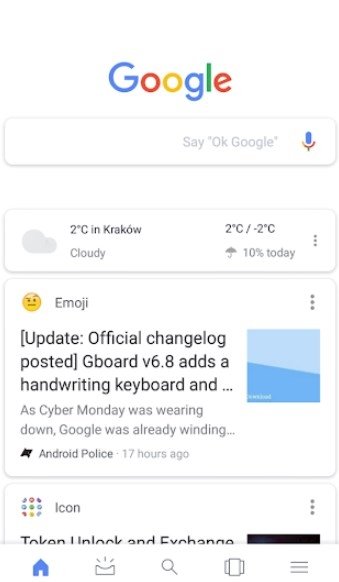This image is a screenshot from a smartphone, displaying a Google search interface against a white background. At the top center of the screen, the colorful Google logo is prominently displayed with the letters in their characteristic colors: a blue "G", a red "O", a yellow "O", a blue "g", a green "L", and a red "E".

Below the Google logo, there's a search bar with a white background and rounded corners, outlined in gray. Inside the search bar, right-aligned text reads "Okay, Google" in gray, accompanied by a microphone icon where the microphone is blue and the stand is red.

Underneath the search bar is a larger white rectangle with rounded corners, containing a weather widget. On the left side of this widget, there's a gray cloud icon. Next to the cloud icon, in black text, it displays the temperature in Krakow as "2°C". Below the temperature, in smaller gray text, it says "Cloudy". To the right of the word "Cloudy," there's a gray umbrella icon followed by "10%" indicating precipitation. Above the current temperature, it shows the expected range for the day as "2°C / -2°C". On the far right of this weather widget, there are three small gray dots arranged vertically.

Further down, there is another large white rectangle with rounded corners. Inside this rectangle, there’s an emoji with eyebrows, and next to it, black text reads "Emoji." In the top right corner of this section, there are three gray dots. Below, there is a section of black text accompanying an image that transitions from light blue on top to dark blue on the bottom.